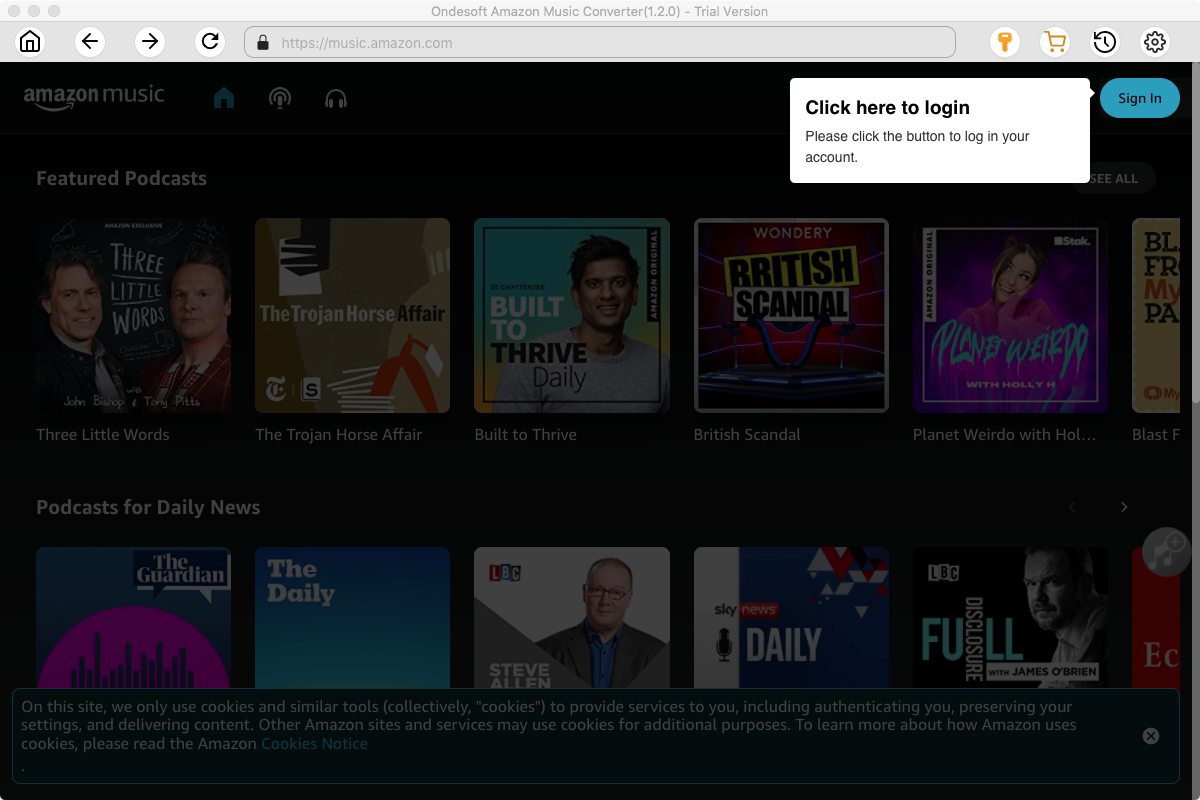The image features the interface of the Ondesoft Amazon Music Converter (version 1.2.0, Trial Version). The top part of the image has a gray and darker gray color scheme with "ONDESOFT Amazon Music Converter (1.2.0/trial version)" displayed prominently. Below this header are four circular icons set against a white background. The first icon on the left is an outline of a black house with a left-pointing arrow beside it. The second icon features a black arrow pointing to the right. The third icon is a refresh button represented by a black circular arrow. 

In the rectangular web browser area below, there is a black padlock icon followed by the URL "https://fastmusic.amazon.com" in gray text. Further down, there are four more circular icons: an Amish key, an Amish card, a black clock, and a black gear. 

The lower section of the image has a black background. On the right side of this section, there's a blue oval button with the text "Sign In" in black. Next to this button, a white square contains the instructions "Click here to log in" in black text, with additional direction to "Please click the button to log into your account."

The bottom part of the image provides a glimpse into various available content on Amazon Music, including podcasts and shows such as "Podcast Three Little Words," "The Trojan Horse Affair," "Built to Thrive," "British Scandal," "Planet Widow with HOL...", "Blast," and more. Some of the listed podcasts are "Daily News," "The Guardian," "The Daily," "Steve Allen," "Daily Sky News," and "Full Disclosure with James O'Brien."